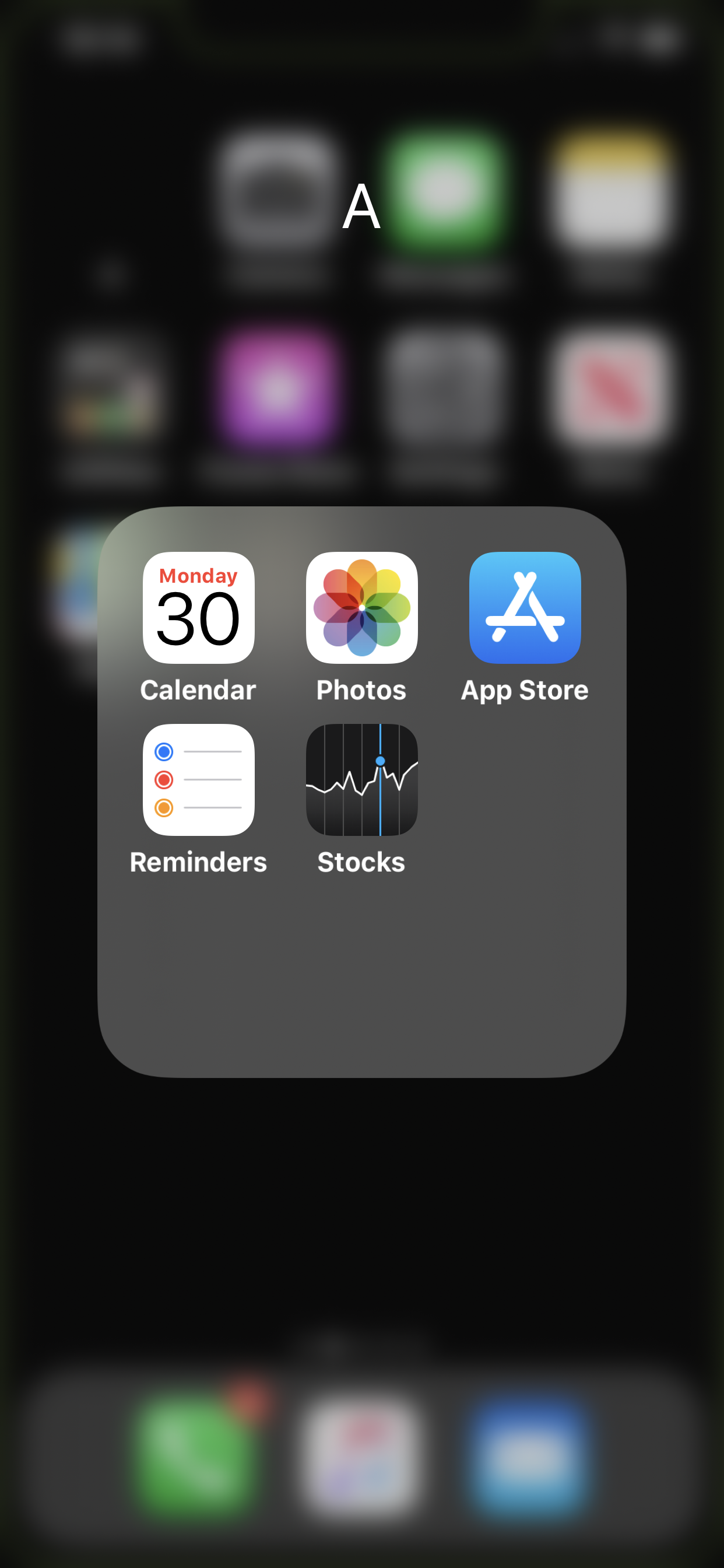A screen capture displays a cell phone's interface, prominently featuring a window with five distinct app icons, sharply in focus, against a blurred desktop background. The first icon is a calendar marked with "Monday 30," indicating a specific date. Beside it is a "Photos" app, represented by a vibrant color wheel. Next is the "App Store" icon, designed as an 'A' constructed from Popsicle sticks, followed by the "Reminders" app, depicted as a classic to-do list. The final icon is for "Stocks," showcasing an up-and-down graph with a notable dot on one of its peaks and a line cutting through it. The backdrop features blurred apps, maintaining focus on the open icons. Dominating the top of the image is a large, capital letter 'A,' suggesting the image may be part of an instructional guide or tutorial.